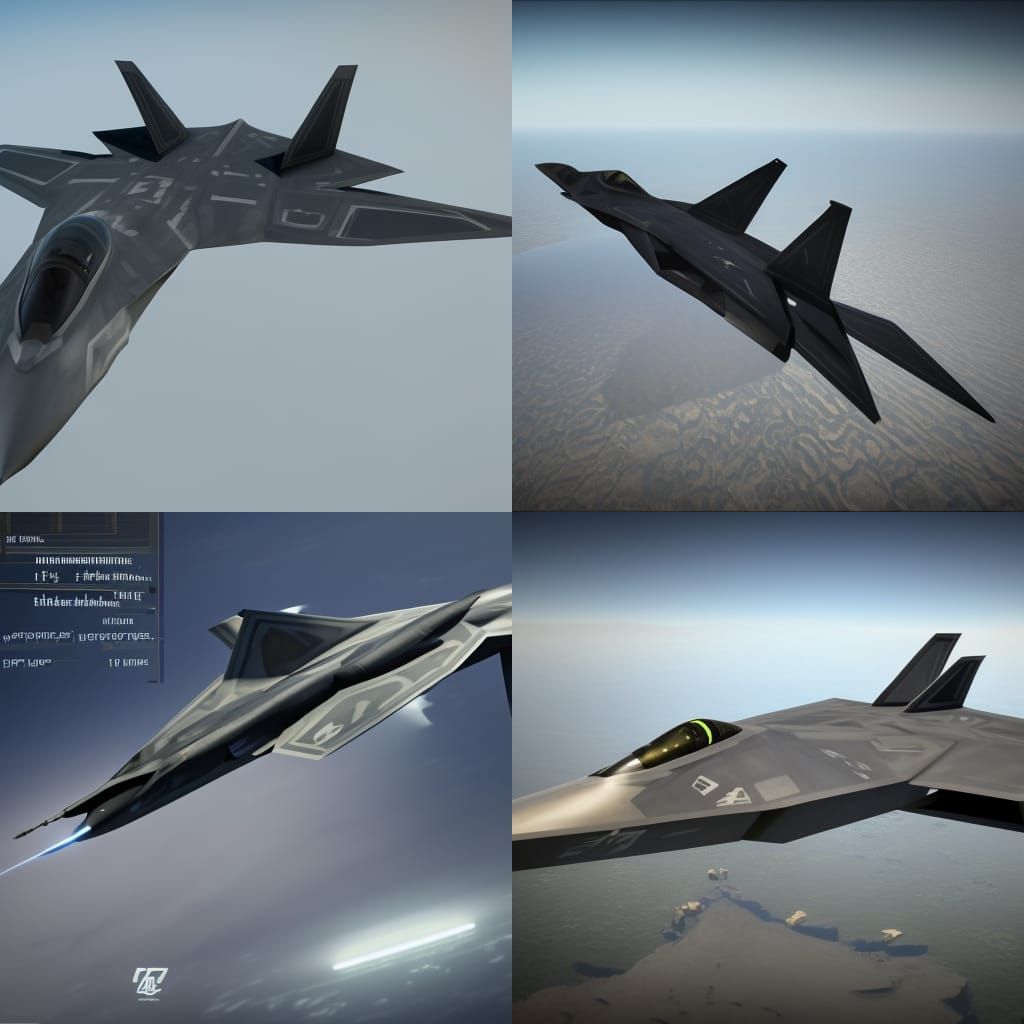This image is a composite of four pictures showcasing a sleek and advanced fighter jet in flight from various angles. The jet has a distinctive grey body with intricate design patterns and two tail fins forming a V shape. Each picture captures the jet in a different context:

1. **Top Left Panel:** The jet is captured mid-flight against a clear, light blue sky, highlighting its aerodynamic structure and dark, tinted cockpit.
2. **Top Right Panel:** This picture shows the jet ascending in a vertical lift, with a ground area in muted brown tones visible below.
3. **Bottom Left Panel:** A detailed shot featuring part of the ground and sky, this image includes textual specifications and a vivid blue flame emitting from the jet's engine, underscoring its power.
4. **Bottom Right Panel:** The jet is shown flying above a landscape featuring an island surrounded by water, with both the sky and ground in the background, providing a scenic overview.

Despite some variations in the jet's appearance across the images, the cohesive display focuses on the jet's design, technological sophistication, and contextual backdrop, combining to give a comprehensive view of this impressive aircraft in action.